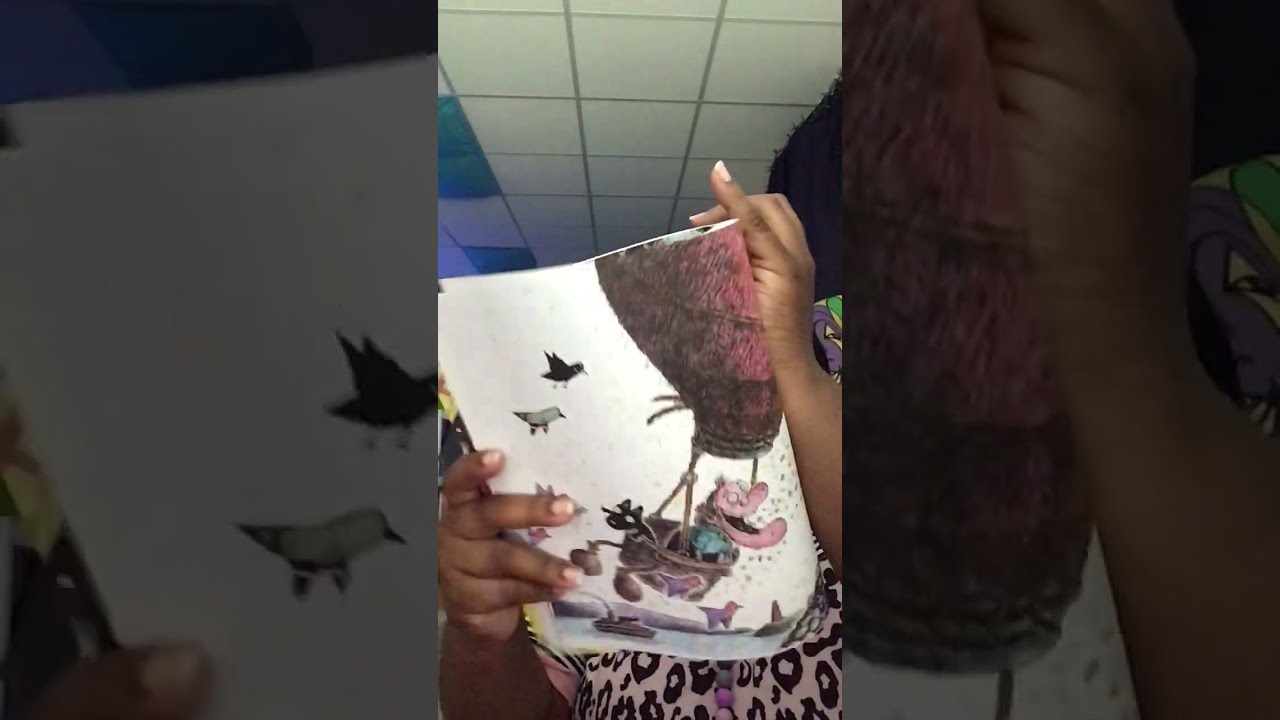The image appears to be a screenshot from a video, presented in a vertical format. It features a black woman, possibly a teenager, whose face is obscured by the book she is holding. Her hands, adorned with a pink shirt featuring black leopard print and a bead necklace in shades of black, gray, dark pink, and light pink, grasp the book. The book resembles a children's book or a magazine and showcases a highly detailed, cartoon-style illustration on the back page. The illustration depicts an old woman laughing in a basket of a red hot air balloon, accompanied by a black cat attempting to climb out. Birds are flying around them in the sky. The setting might be a classroom, indicated by the white tiled ceiling visible in the background.